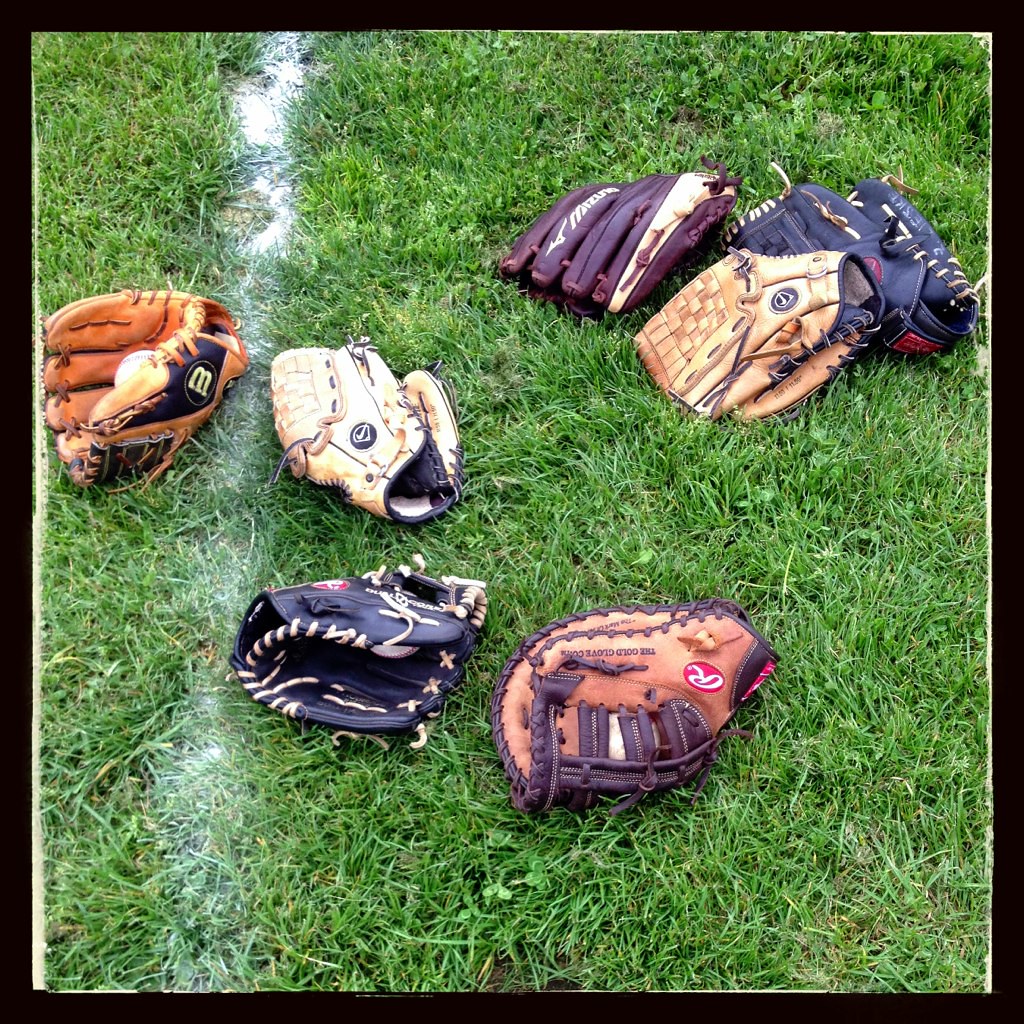This square Instagram-style photograph, framed by a thick black border, captures an assortment of eight baseball gloves spread out on short, uniform green grass, dotted with small patches of clover. The gloves exhibit a variety of styles and colors, including maroon, tan, beige, black, bright buckskin, and pale shades. Some gloves feature dark brown trimmings, while others have distinct black and white leather detailing. Positioned along the left side of the image, a white chalk line runs vertically, slightly diagonal, further adding a dynamic element to the composition. A subtle yellow filter overlays the image, enhancing its warm tones without compromising the authenticity of the colors. The gloves are arranged with three clustered in the upper right, two pairs close together, and the remaining scattered more centrally and near the lower part of the frame.